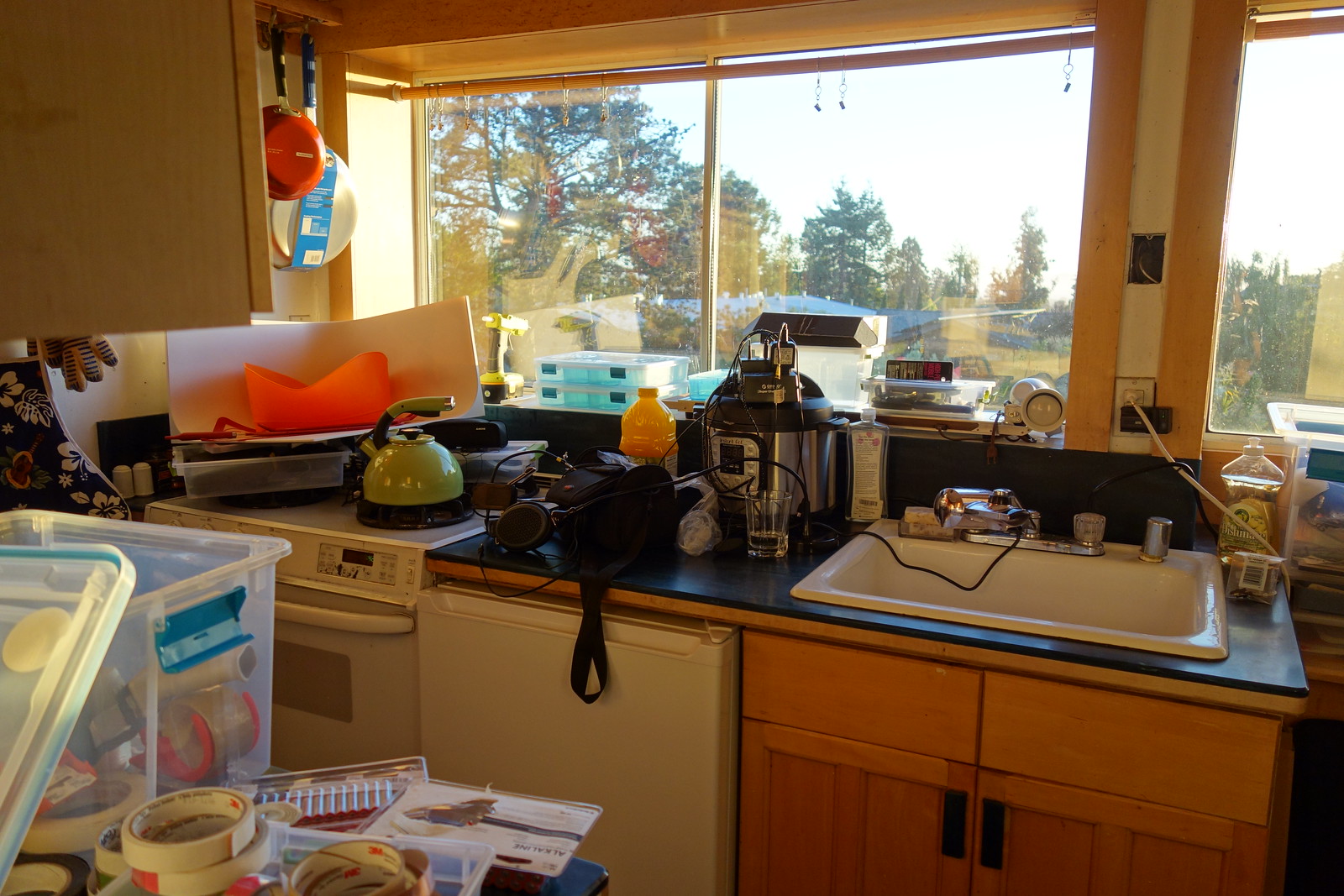The image depicts a cluttered kitchen scene. On the black countertop, a variety of items are strewn about, including a pressure cooker, a kettle, a bag, and a carton of orange juice. To the right side of the photo, there's a white sink built into the countertop, with tan-orange wooden cabinets underneath. Adjacent to the sink on the same counter space is a dishwasher. Further to the right, there's a white stove with an oven, and above it, two pans are hanging from a mounted display or the ceiling. In the background, large windows offer a view of trees outside, adding a touch of nature to the otherwise busy kitchen interior.